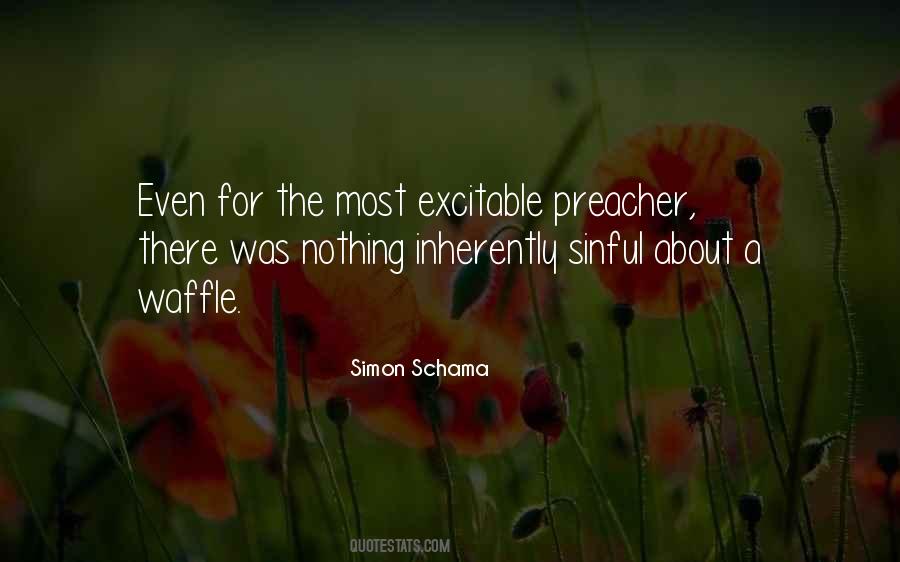The image features a digital artwork with a blurred outdoor setting of flowers and greenery in the background. Prominently displayed in the center is a white text quote: "Even for the most excitable preacher, there was nothing inherently sinful about a waffle." The quote is attributed to Simon Schama and is followed by the website name, Quotestats.com, just below the attribution. The background showcases a mix of red and orange flowers, along with some flowers that have yet to bloom, set against a blurry green backdrop resembling grass and leaves. The overall composition gives the appearance of an inspirational quote sign hosted on Quotestats.com.